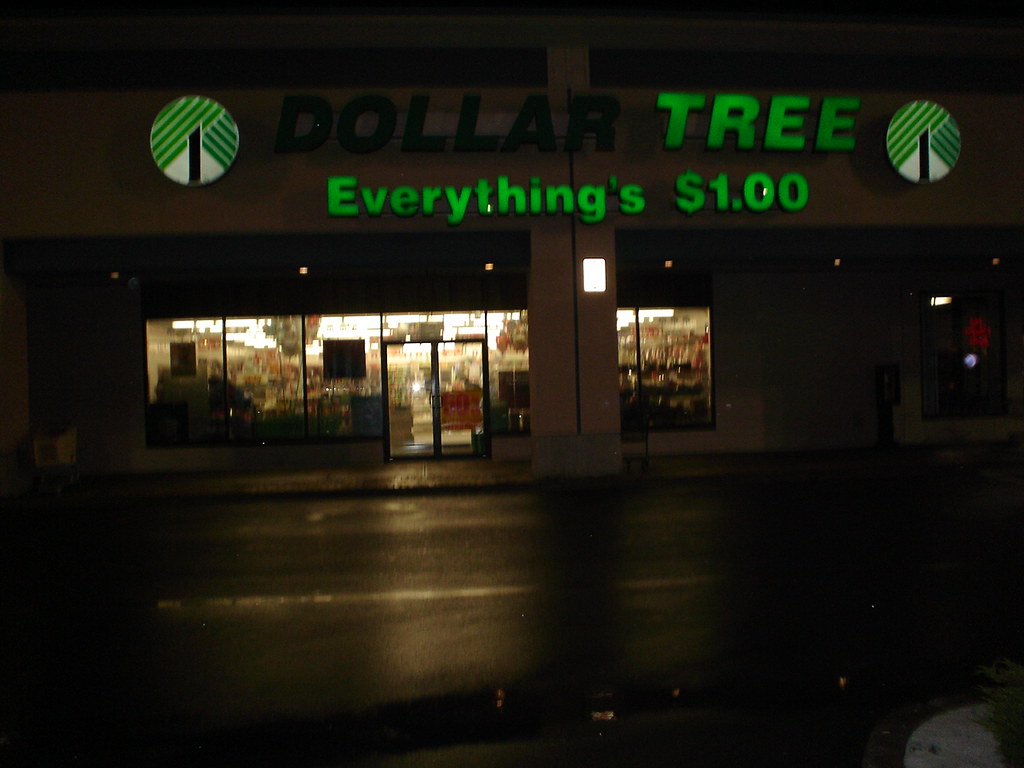This nighttime photograph captures the exterior of a Dollar Tree store. The "Dollar" portion of the store's illuminated sign is unlit, rendering it black, while the "Tree" remains brightly lit. Below the store name, an illuminated sign reads "Everything's $1.00." To the left of this signage, there are symbols featuring the number 1, set against a background of green lines. The image is taken at night, highlighting the stark contrast between the brightly lit store interior and the surrounding darkness. The store’s interior is visible through the windows, showcasing aisles filled with various items. Additionally, signs are affixed to the windows, and there is an exterior light mounted on a column, casting a glow onto the scene. The street in front of the store receives a slight illumination from this setup, adding a small pool of light amidst the overall dark atmosphere.